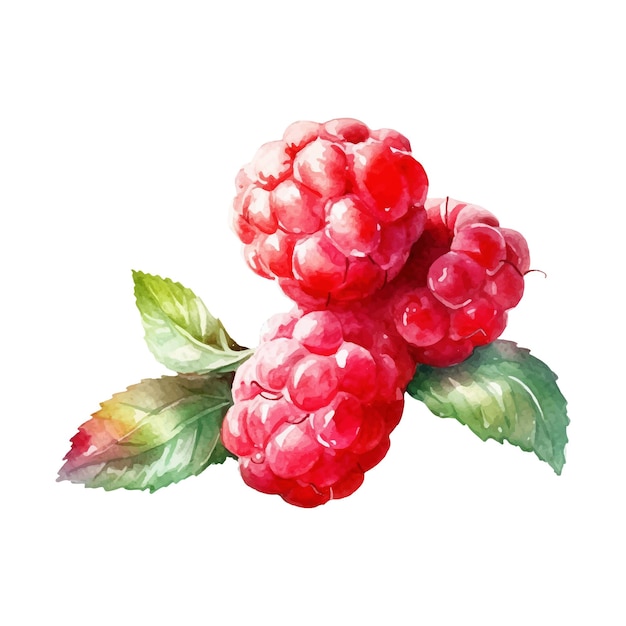This image is a digitally crafted watercolor painting of three vibrant raspberries and three detailed leaves, set against a clean, white background. The raspberries are arranged in an upside-down triangular formation, showcasing their bright pink color with white accents that give a reflective, shiny appearance. You can also notice the fine hair-like structures on the berries and a visible hole at the top of one raspberry. The leaves, curling in different directions, are primarily green, displaying their veins prominently. One leaf on the left has a striking tip with hues ranging from yellow to orange, pink, and purple, adding a colorful contrast. The entire composition is free-floating without any visible stems or plant attachments, emphasizing the vivid details of the berries and leaves.